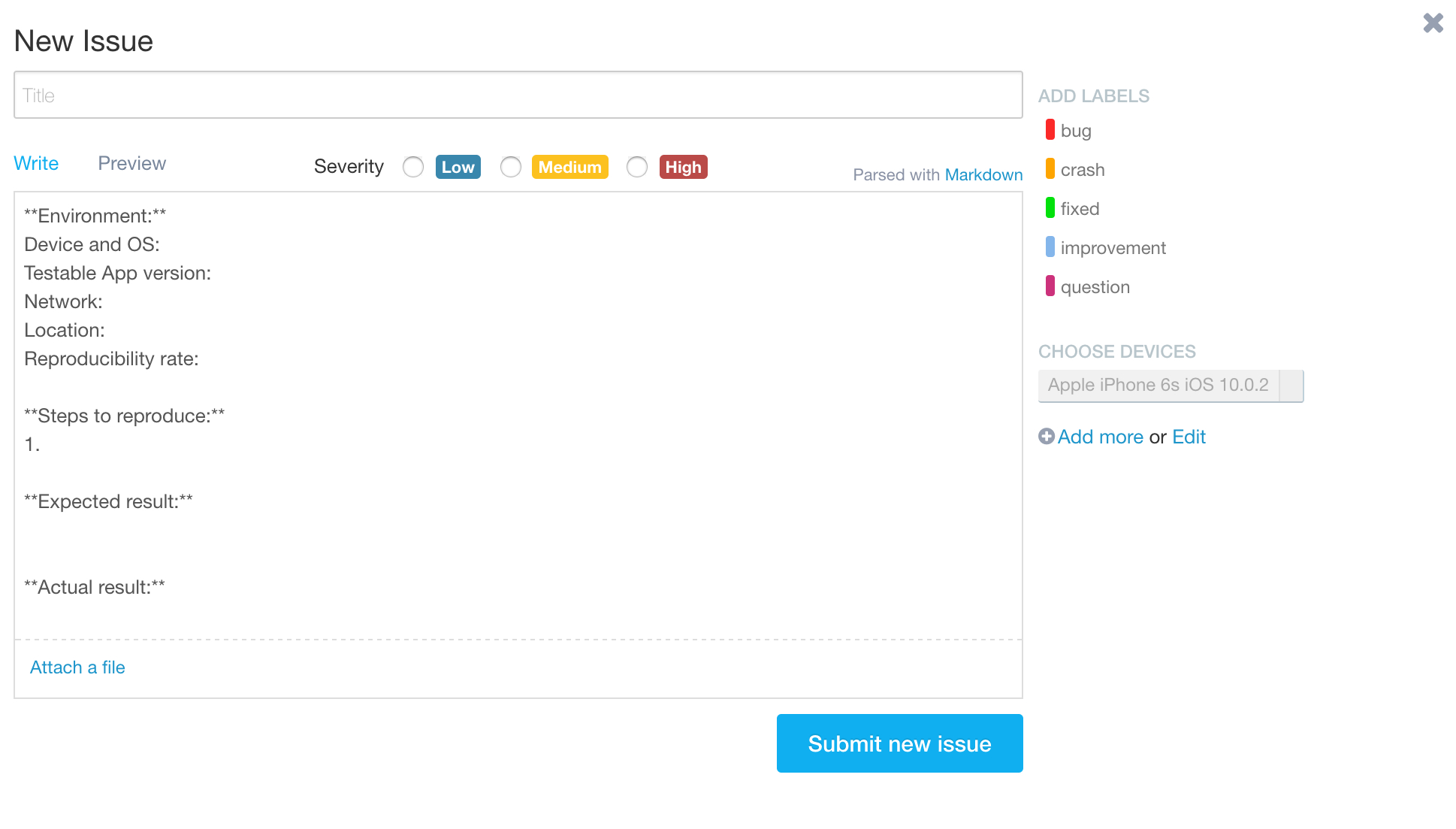In this image, we see a detailed form for submitting a new issue on a platform. The upper left corner of the form contains a section titled "New Issue," and in the upper right corner, there is an 'X' button for closing the form. 

Below this, on the left side, there is a text box labeled "Title," with an option to "Add Labels" at the right end of the text box. The available labels are color-coded: red for "Bug," orange for "Crash," green for "Fixed," blue for "Improvement," and purple for "Question."

Further down, there is a section titled "Choose Devices" with "Apple iPhone 6s iOS 10.0.2" listed. Next to this, there is an "Add More or Edit" button. 

To the left of these options, there's a large text box titled "Write Preview," with buttons to indicate severity levels: Low, Medium, and High. Inside this text box, the following placeholders are provided: "Environment," "Device and OS," "Testable App Version," "Network," "Location," "Reproducibility Rate," "Steps to Reproduce," "Expected Result," and "Actual Result."

At the bottom left of the text box, there is a button labeled "Attach a File." Near the bottom right corner of the text box, there's a blue rectangle button with white text that reads "Submit New Issue."